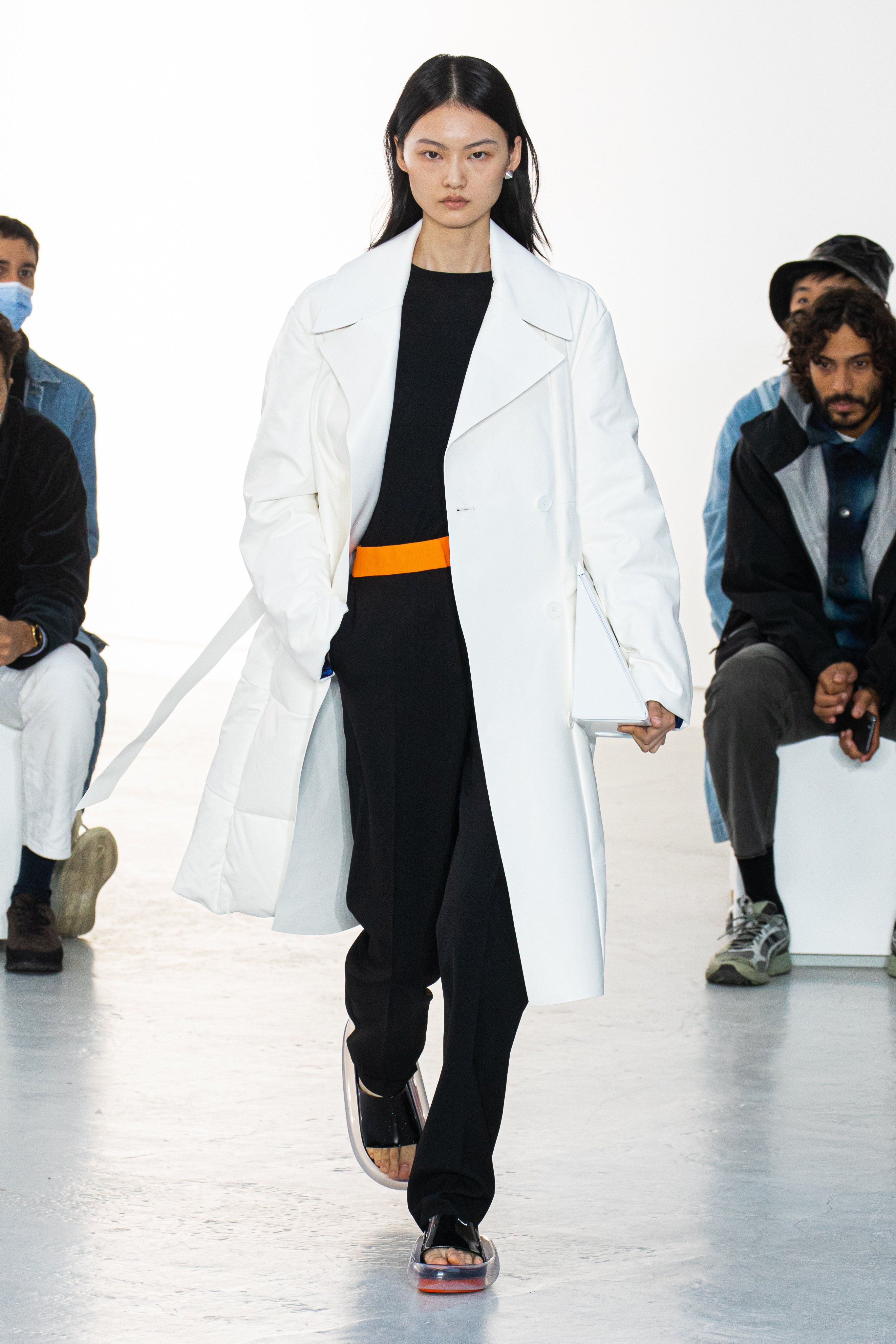A young, pretty Asian woman in her early 20s is modeling on a sleek, glossy runway that features a white backdrop and a shiny, light-colored floor. She has long, black hair parted in the middle and tucked behind her ears. Her outfit consists of a white lab coat-style trench coat that reaches her knees, paired with a black top and black pants. She cinches her waist with a pumpkin orange belt and accessorizes with silver earrings. She carries a triangular purse in her right hand and completes her look with unique flip-flop-style shoes that have black straps over the feet and clear gel-like soles with a reddish hue. The photo captures a vibrant fashion show scene with seated observers on both sides, including a few notables: an Indian man with a mustache and bucket hat, a younger man in a blue face mask and jean jacket, and a woman with black socks and brown shoes. The model walks confidently, maintaining a serious expression with light lip gloss highlighting her natural beauty.